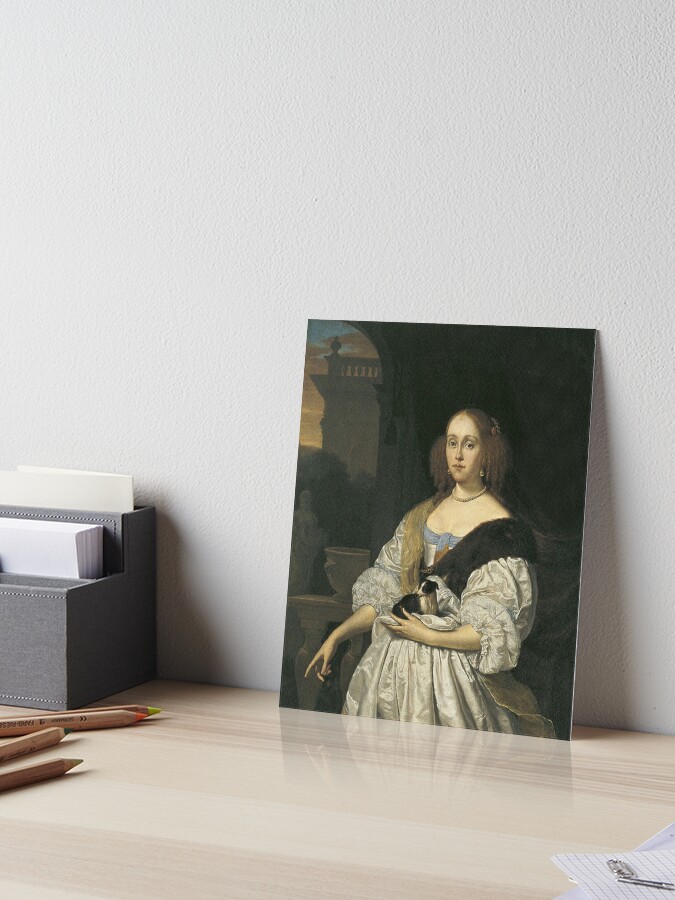The image depicts a small rectangular painting, slightly taller than it is wide, approximately the size of a postcard or a few business cards. This unframed reproduction of a Victorian-style portrait shows an old-fashioned, elegantly dressed woman in a puffy, flowing dress with a little dog in her lap and her other arm hanging down. The painting is leaning against a slightly off-white, light gray, textured wall. It is situated on a glossy, light-colored wooden surface that reflects part of the painting. To the left of the painting, there's a gray box likely used for holding stationery, accompanied by a set of wooden colored pencils. Further to the left, there are vertical files with papers sticking out. On the right-hand side of the scene, we see some note paper with paper clips. The overall setting suggests a work area or desktop.